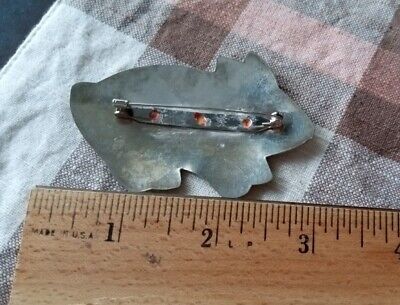In this color photograph, the back of an oxidized metal pin or brooch, shaped like a small animal, is prominently displayed. The pin features discernible aspects of an animal, such as a tail, face, ears, and feet, and is steely gray or rusted in appearance. Attached to the back of the animal-shaped metal is a clothespin or a safety pin, seemingly glued or welded in place, for fastening to clothing. The object rests on a checkered tablecloth with light brown, dark brown, and white patterns. At the bottom of the image, a wooden ruler, marked with measurements and labeled "Made in the USA," stretches up to four inches, indicating the pin itself is around two to three inches in length. The background captures both the textured tablecloth and the contrasting, darker hues beyond its edges.